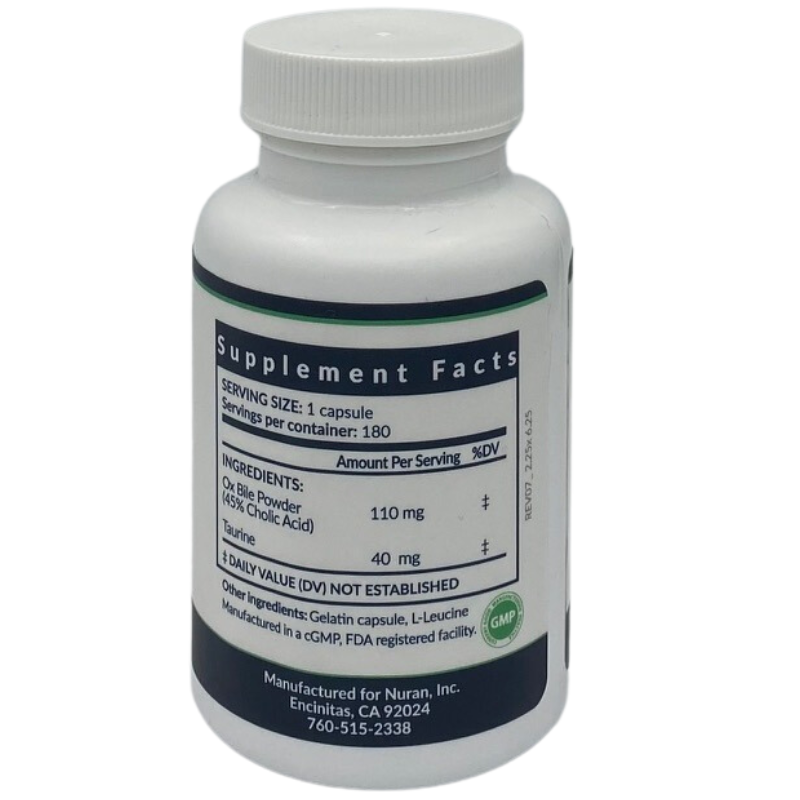This image shows a white medicine bottle with a matching white twist cap. The bottle is adorned with a detailed label on the back. The top of the label features a bold black bar with a thin green underline beneath it. Prominently in the center, the label reads "Supplement Facts." The text below this outlines the supplement information: "Serving Size: 1 Capsule" and "Servings Per Container: 180." Another darker line separates this from the "Amount per Serving" and "percent DV" information. 

The primary ingredients listed are ox bile powder, specified as 45% colic acid, with an amount per serving of 110 milligrams. This is followed by taurine at 40 milligrams. Both ingredients feature a symbol indicating that the daily value is not established. Other listed components include a gelatin capsule and L-leucine, with a note that the product is manufactured in a CGMP FDA-registered facility. There's also a green circular seal with the letters "GMP" confirming this compliance.

At the bottom of the label, in a black bar, it states: "Manufactured for Nuran Inc., Encinitas, California, 92024," followed by the contact number "760-515-2338".